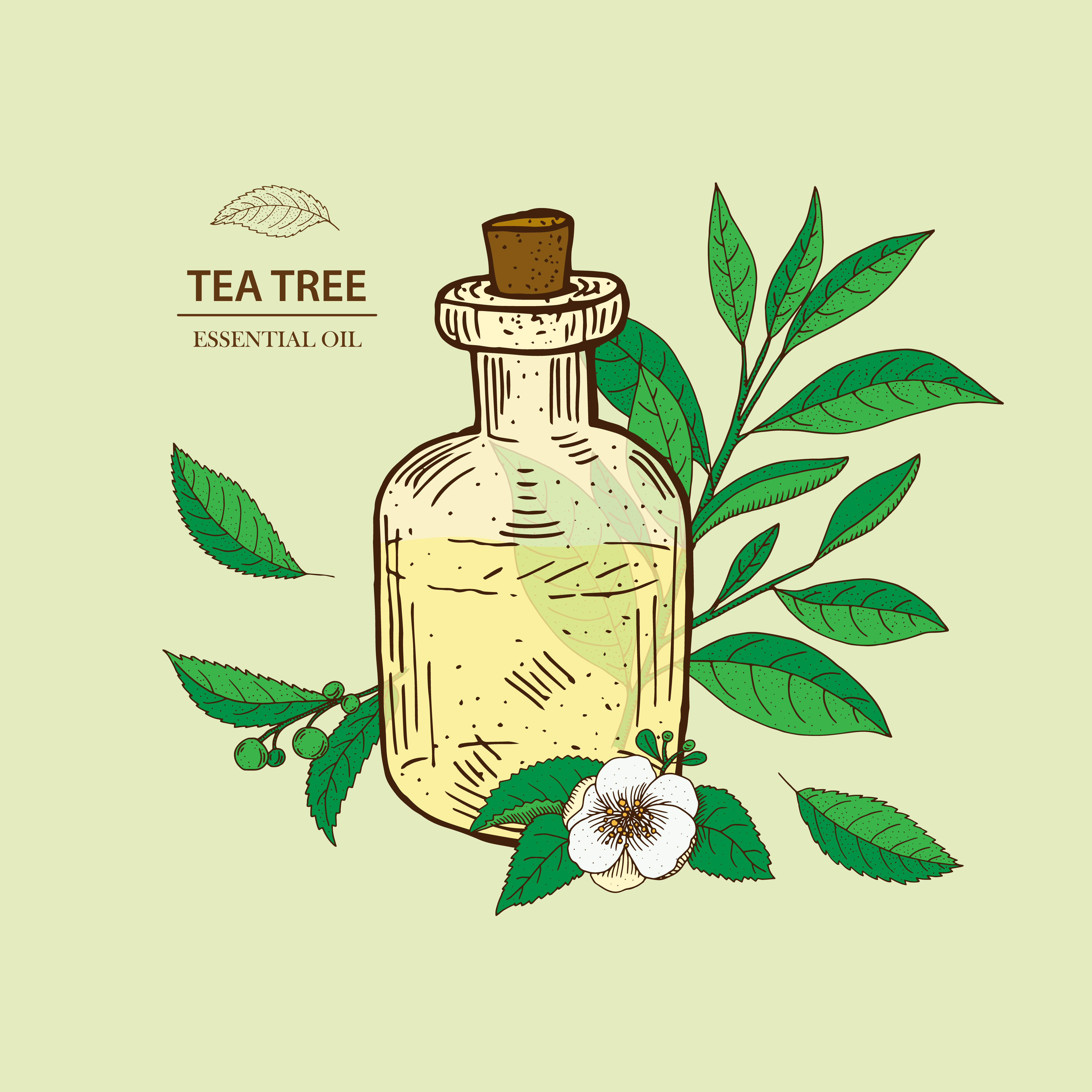The image appears to be a meticulously designed, computer-generated promotional illustration for tea tree essential oil. Set against a very light green background, the left side of the image features a small brown drawing of a tea leaf with the text "tea tree" written in brown, underlined, followed by "essential oil" also in brown. Dominating the upper central portion, there is a vintage-style brown glass bottle with a thick cork stopper, filled about 75% with a light yellow liquid. The bottle has intricate brown etch markings and lines around it, enhancing its classic appearance. Surrounding the bottle are vibrant green leaves and a small, central white flower. At the bottom, green leaves along with scattered small green berries extend towards the right side, adding to the botanical theme. This detailed and aesthetically appealing advertisement likely aims to showcase the tea tree essential oil product.